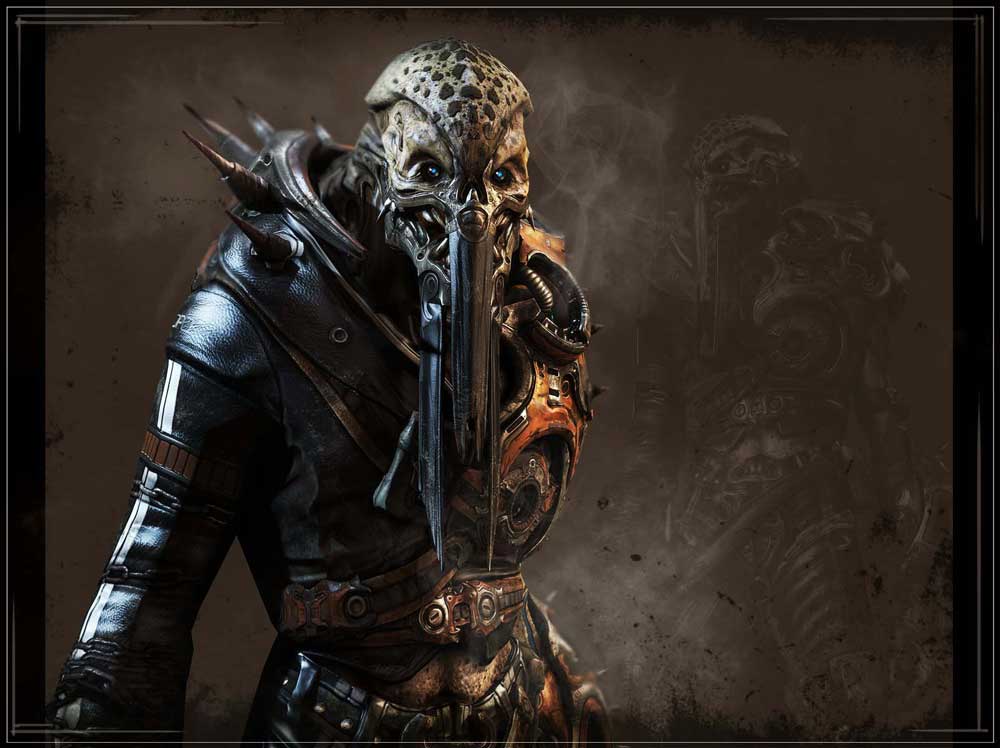The image depicts a menacing, alien-like creature that appears to be from a video game or fantasy world. The creature, resembling a cryptid, has a silver, metallic head with dark black, beady eyes and a nose that extends past its chest, resembling a long, sharp sword. Its mouth is filled with sharp, jagged teeth like those of a piranha. The head features a distinctive spotted pattern and the chin and jaw are adorned with additional sharp protrusions. The creature is clad in a dark, metal-colored bodysuit accented with brown outlines, featuring a spiked collar and armor. It wears a black jacket with a brown stripe around the upper arm, a brown belt, brown pants, and another black belt. The background is predominantly dark with smoke and shadows. To the right, a shadowy profile of the same creature blends into the smoky, grayish-white background, providing a haunting, mirrored silhouette of the creature.